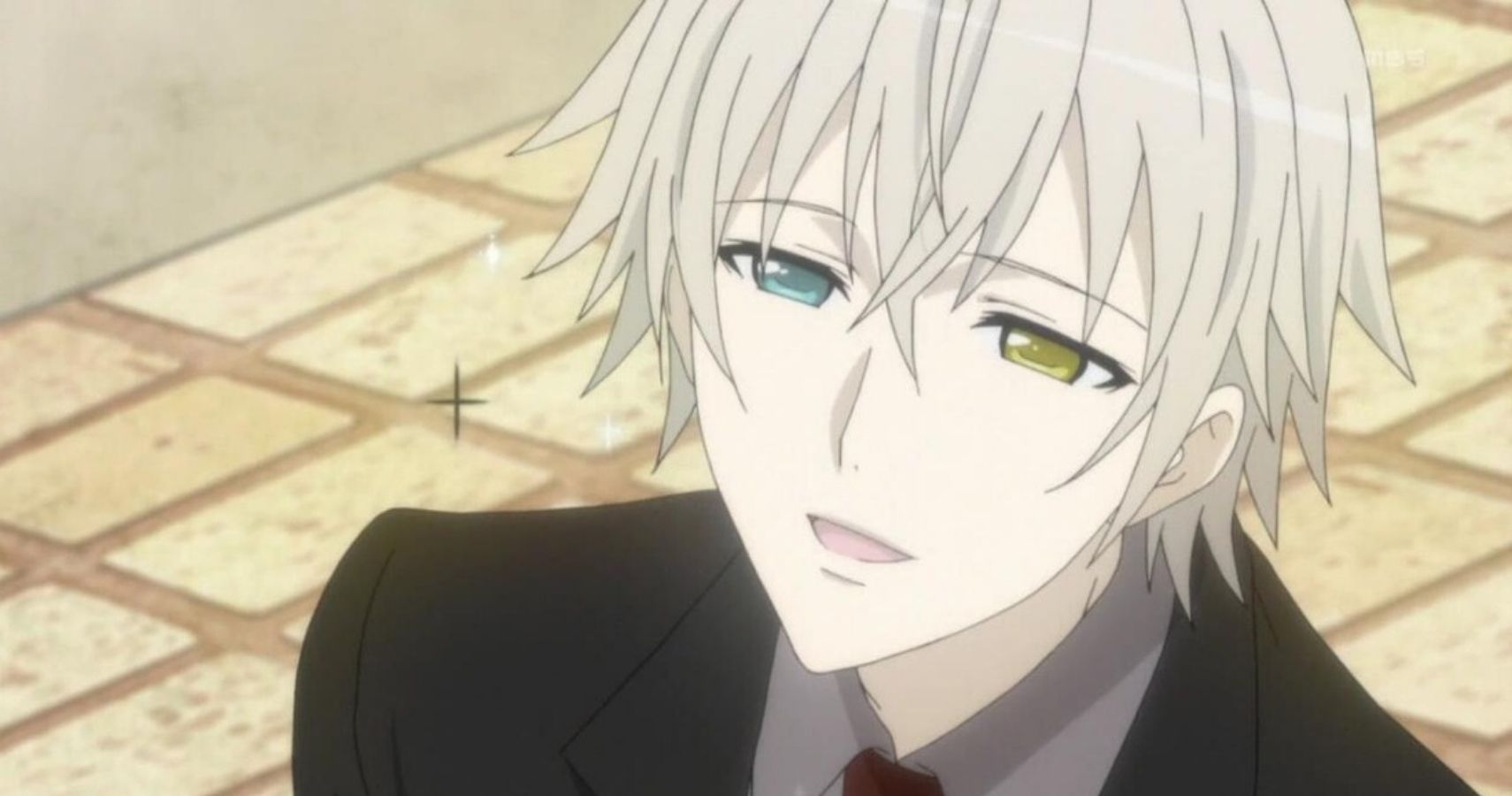This image depicts a character in an anime style, standing on the right side of the frame. The character has very pale skin and distinct facial features, including a pointed chin, small pink lips, a very small nose, and wide eyes with flat bottoms. The left eye is a striking aqua blue, while the right eye is a unique blend of mustard yellow with a green tinge. Their shaggy, chin-length hair is light gray, almost white, and falls across their face in forks. 

The character is dressed in a black suit jacket over a gray collared shirt and a maroon tie that peeks out from between the collars. They are standing on a slightly blurred tiled floor with pale yellow to beige tiles and brown grout. In the background, there is a concrete wall with a light brownish taupe color. The concrete wall curves slightly and comes up in the top left of the frame. The character is looking up and to the left, with their mouth slightly open, as if they are speaking, adding a sense of action to the scene. There is no text present in the image.